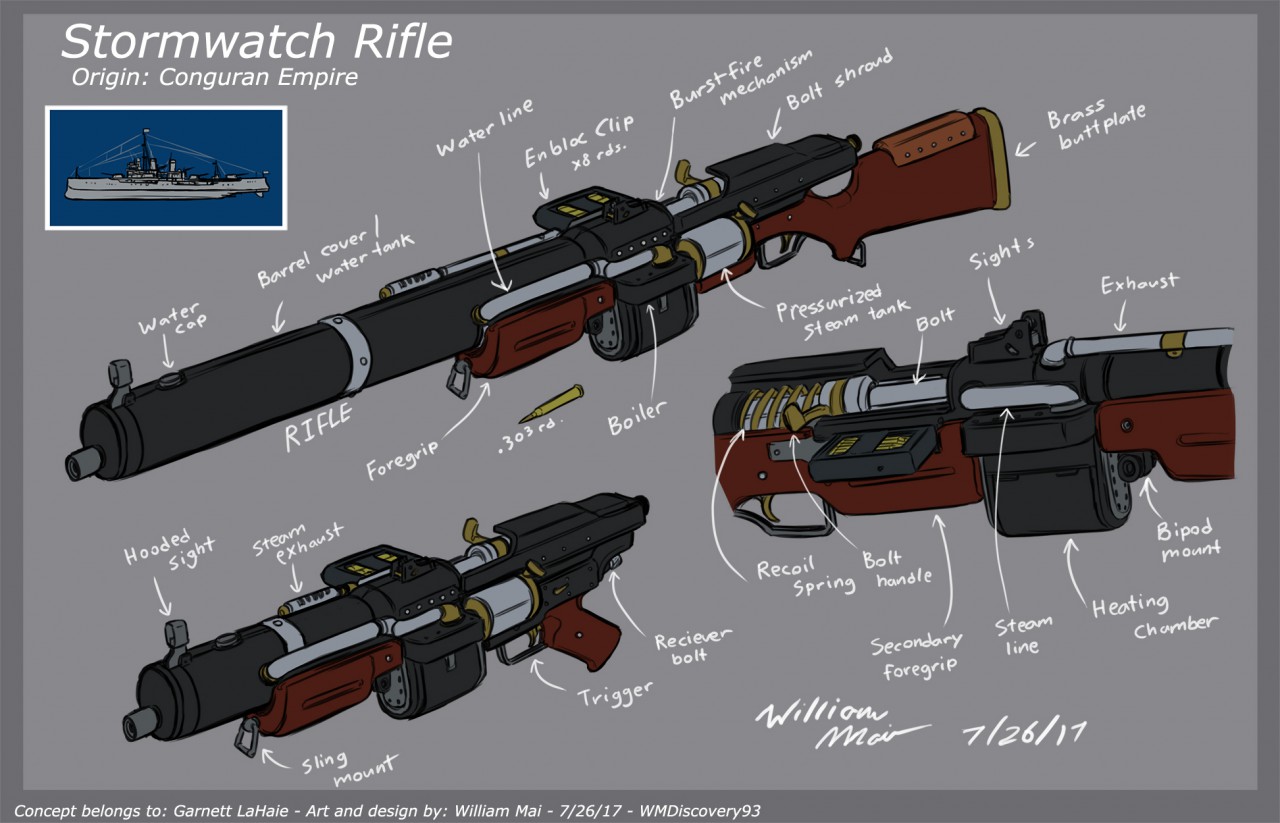This detailed artwork showcases the Storm Watch Rifle, originating from the Konguran Empire, against a solid gray background with a darker, grayer border. In the top left corner, the title "Storm Watch Rifle, origin Konguran Empire" is prominently displayed in white. Adjacent to this is a small blue rectangle featuring a silver ship. The rifle is meticulously labeled with numerous parts identified by arrows and text, including significant components such as the water cap, barrel cover, water tank, water line, M-block clip with eight rounds, burst fire mechanism, bolt shroud, brass butt plate, pressurized steam tank, boiler, and the .303RD bullet. Additional features labeled are the foregrip, head sight, steam exhaust, receiver bolt, trigger, and sling mount. Included in the artwork, text at the bottom credits Garnet LeHay with the concept and identifies William Mai as the artist and designer, dated 07/26/17 under the tag WM Discovery 93.